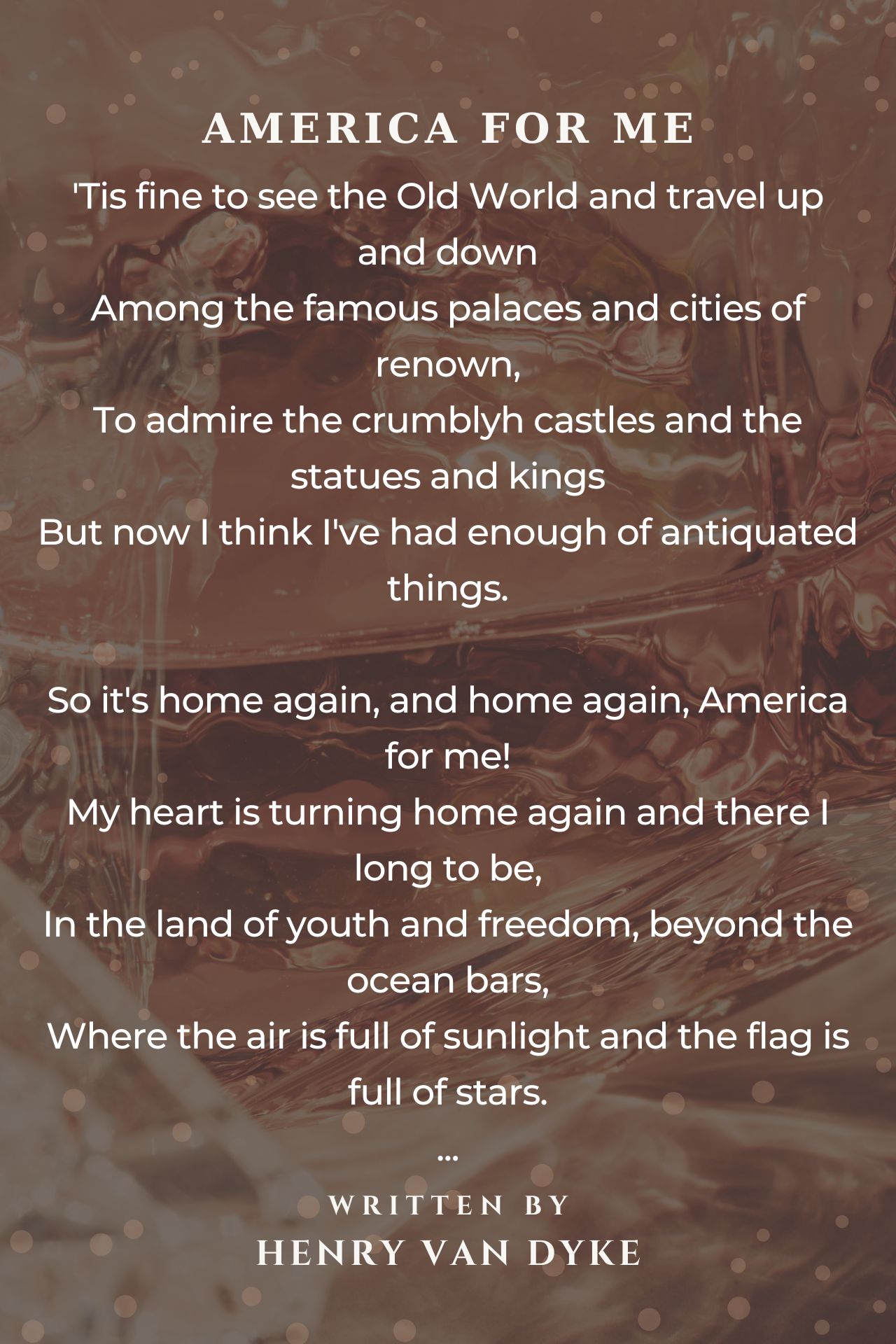The image is a poster featuring the lyrics to a song or poem entitled "America For Me," written by Henry Van Dyke. The text is presented in white, uppercase, bold letters, prominently displaying the title at the top. The verses go, "'Tis fine to see the old world and travel up and down among the famous palaces and cities of renown, to admire the crumbly castles and the statues of kings, but now I think I've had enough of antiquated things. So it's home again and home again, America for me. My heart is turning home again and there I long to be in the land of youth and freedom beyond the ocean bars where the air is full of sunlight and the flag is full of stars." At the bottom, it is credited with "Written by Henry Van Dyke." The background is brown with scattered circles in varying shades of the same palette, possibly depicting a faded, patriotic scene that includes an American flag. The visual elements in the background are blurred and subtle, ensuring the focus remains on the text.